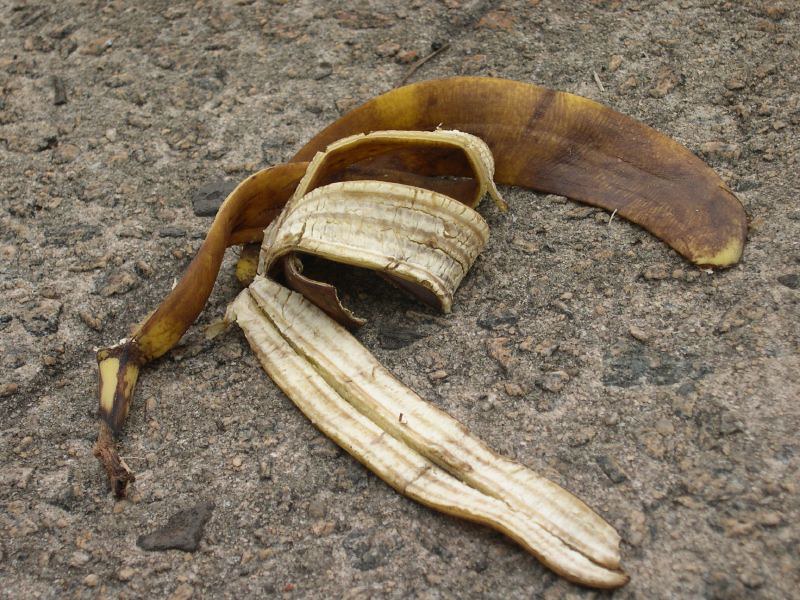This photograph captures a discarded banana peel lying on a textured sidewalk surface. The peel shows signs of aging and decay, indicating the banana was very ripe when it was peeled. The inside of the peel has not fully darkened, suggesting it was recently exposed. Conversely, the exterior of the peel is starting to rot and turn black. The sidewalk consists of large, gray pavers with a visible expansion joint that runs diagonally through the image, designed to prevent the concrete from cracking. This small gap between the pavers allows for expansion and contraction due to environmental changes. The detailed, tactile surface of the pavers contrasts with the organic, deteriorating banana peel, highlighting the interaction between natural waste and urban environments.